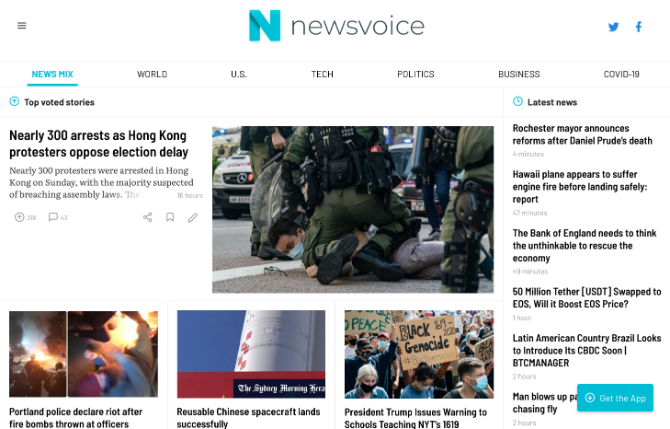This image, sourced from the website Newsvoice, showcases the main interface of the platform. Prominently displayed in the upper center is the Newsvoice logo, which features a bold "N" positioned to the left of the site's name, though center-justified overall. 

Dominating the screen is the primary navigation menu running horizontally across the top, offering options such as News Mix, World, U.S., Tech, Politics, Business, and COVID-19. Directly beneath this menu on the left side, the section labeled "Top Voted Stories" is highlighted. 

The main story, occupying a significant portion of the page, is headlined "Nearly 300 Arrests as Hong Kong Protestors Oppose Election Delay." To the right of this headline, a poignant image captures the dramatic moment: a person is lying on the ground with several military personnel surrounding and restraining them, vividly illustrating the tensions and confrontations occurring.